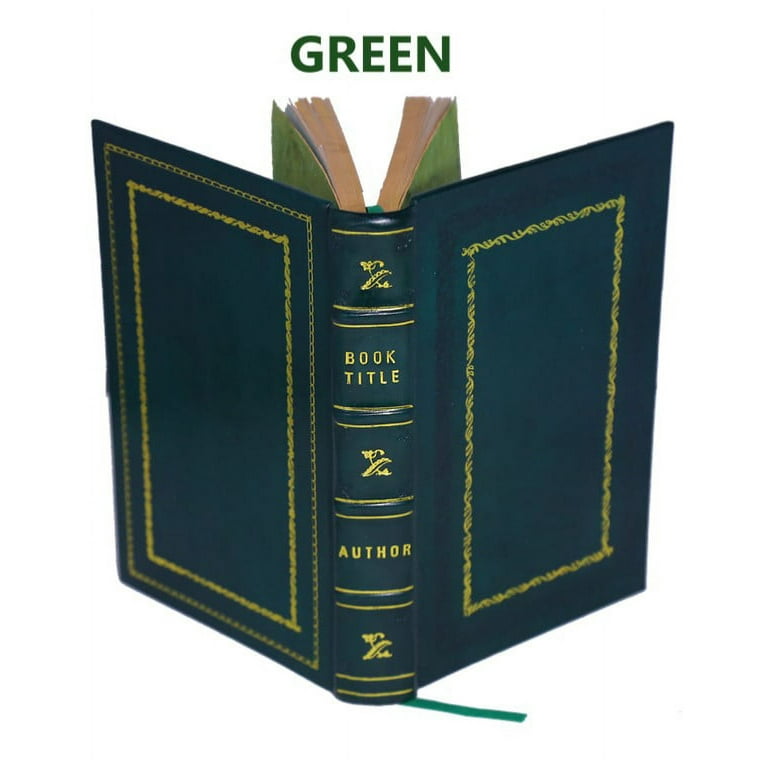The image features an open book with its pages facing away from the viewer, revealing the front and back covers along with the spine. The book has a rich forest green cover adorned with gold accents. Both the front and back covers are framed by a gold border, with the back cover featuring an additional outer gold border, creating a double-frame effect. The spine of the book is detailed, displaying the title "BOOK TITLE" in all capital letters, followed by the word "AUTHOR" slightly further down. Notably, the spine also includes three identical gold symbols. A ribbon bookmark emerges from the spine and drapes over the center of the pages. Above the book, the word "GREEN" is vividly displayed in green capital letters, adding a final touch to the composition.